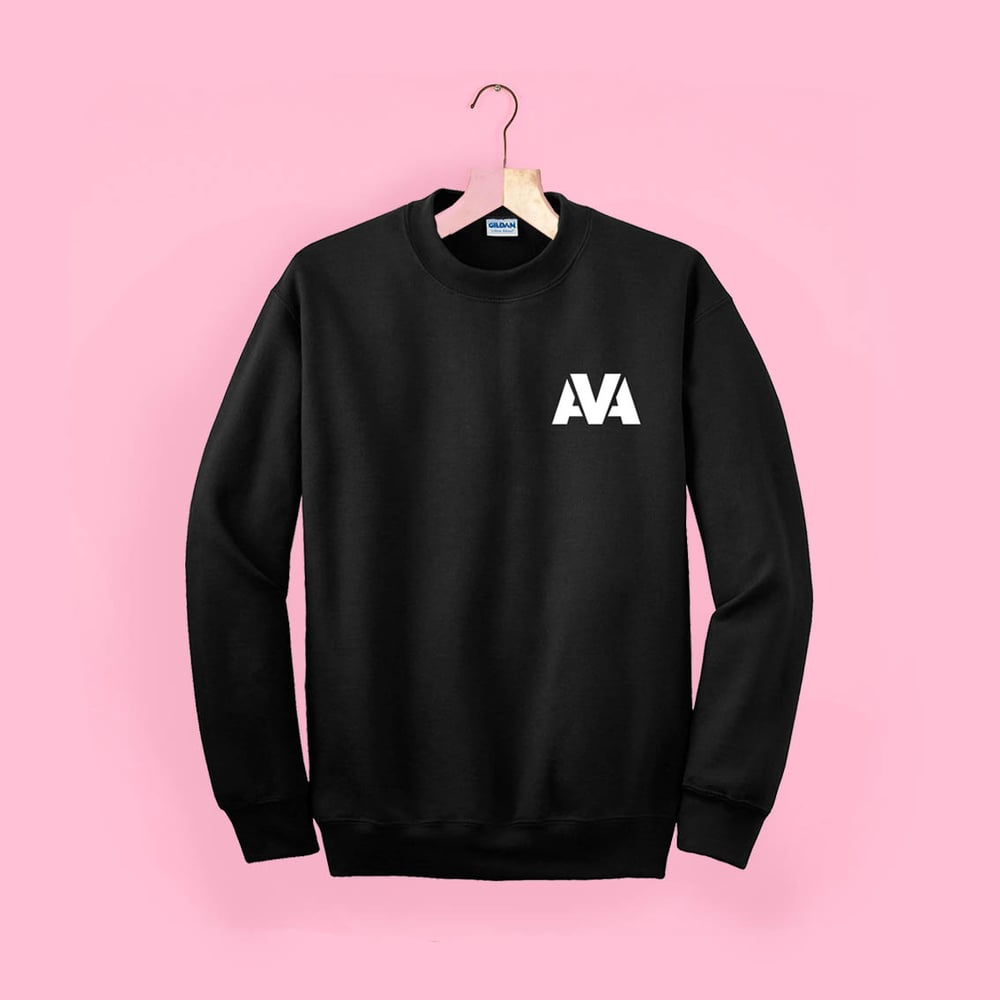This image depicts a black sweatshirt hanging on a clothes hanger against a vibrant pink background. The hanger itself is distinctive, featuring a two-toned design: pink on the left side and light tan wood on the right, with a dark brown metal hook at the top. The sweatshirt, which has elastic cuffs at the sleeves and the bottom hem, displays the letters "AVA" on the upper left chest area in white. A tag inside the sweatshirt reads "Gildan" in blue on a white label, indicating the brand. The overall scene is brightly lit, highlighting the contrast between the dark sweatshirt and the pink backdrop.